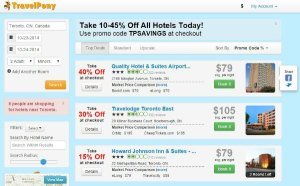The image showcases a screenshot of a website called "Travel Pony," with a yellow logo featuring a small horse beside the text. The background of the website is a light blue color. At the top of the screen, there is a search box where users can input their travel dates and information. Below this, a prominent yellow button is available for interaction.

In the middle of the screen, there is a long, skinny pink rectangle. Lower down, there is a clickable teal rectangle that says "View More." The website promotes a special offer with the text, "Take 10 to 45% off all hotels today," and instructs users to use the promo code "TP Savings" at checkout.

Further details on the page include three hotel options:
1. The first section offers 40% off at checkout, priced at $79 per night, with a green button to click.
2. The second option offers 30% off at checkout, priced at $105 per night, also featuring a green button.
3. The final option provides 15% off at checkout, also priced at $79 per night, with a corresponding green button for user action.